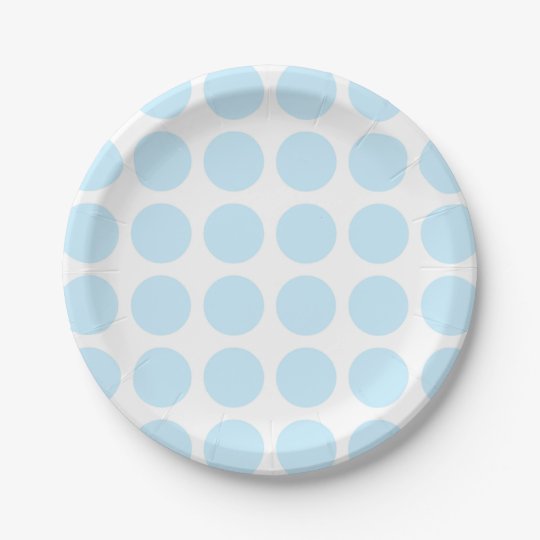This image features a simple yet elegant white paper plate adorned with neatly arranged, powder blue polka dots. These polka dots, organized in six precise rows both vertically and horizontally, create a harmonious and classy pattern against the white, slightly eggshell-toned background of the plate. The edges of the plate exhibit subtle crinkles, characteristic of its upward curving sides, adding a touch of texture to the otherwise smooth surface. The photo is centered on the plate, presenting it as a perfect round circle without any text or additional elements, highlighting the plate’s understated sophistication.